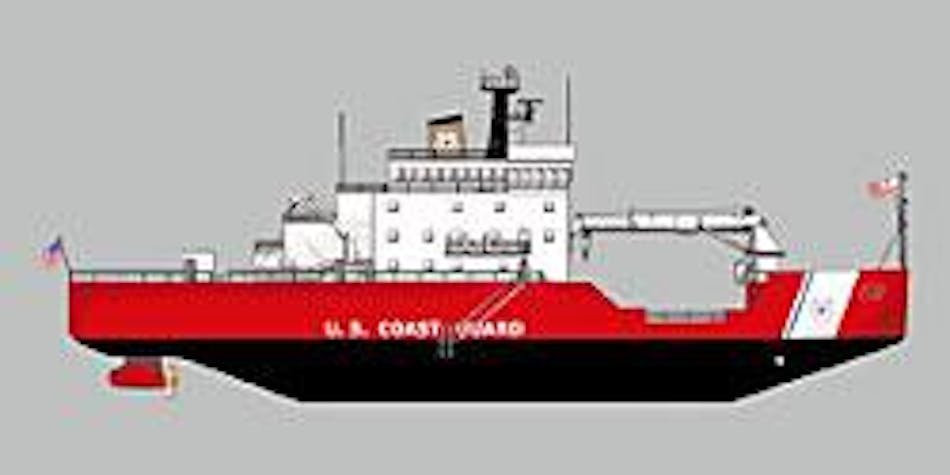This blurred and slightly pixelated illustration depicts a U.S. Coast Guard ship against a light gray background. The ship features a black hull with a prominent red and white striped diagonal section along its side. The upper structure of the vessel is primarily white with small square windows and includes a tall black instrument tower, likely equipped with radar or sonar systems. The deck area appears open with railings along the front, suggesting it might be designed for launching and recovering a submersible vehicle. The ship is adorned with the "U.S. Coast Guard" insignia in white letters prominently displayed on the red section of the hull. An American flag is flying at the stern of the vessel. Additionally, there's mention of a red rudder at the front and crane-like machinery mounted at the back. Despite the image's poor quality and visible JPEG artifacting, these details help identify it as a detailed representation of a U.S. Coast Guard ship.